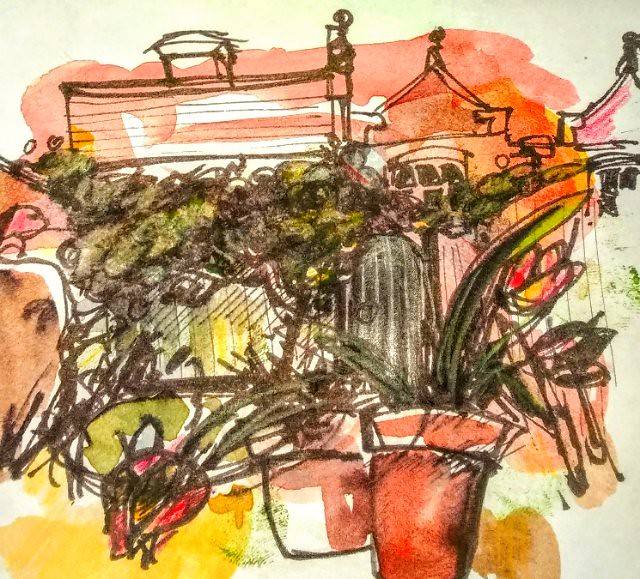This image is a detailed drawing, potentially created using either watercolor, colored ink, or magic marker. In the foreground, positioned towards the left and stretching into the lower right-hand corner, there is a plant pot containing a green spider plant, distinguishable by its long, narrow leaves. Adjacent to it is a significantly larger pot housing a plant that resembles a small tree. In the background, a series of house rooftops can be seen, adding to the somewhat chaotic composition of the drawing. Additionally, in the lower left-hand corner, there is a sketchy depiction of a red insect, adding an intriguing, whimsical touch to the scene.